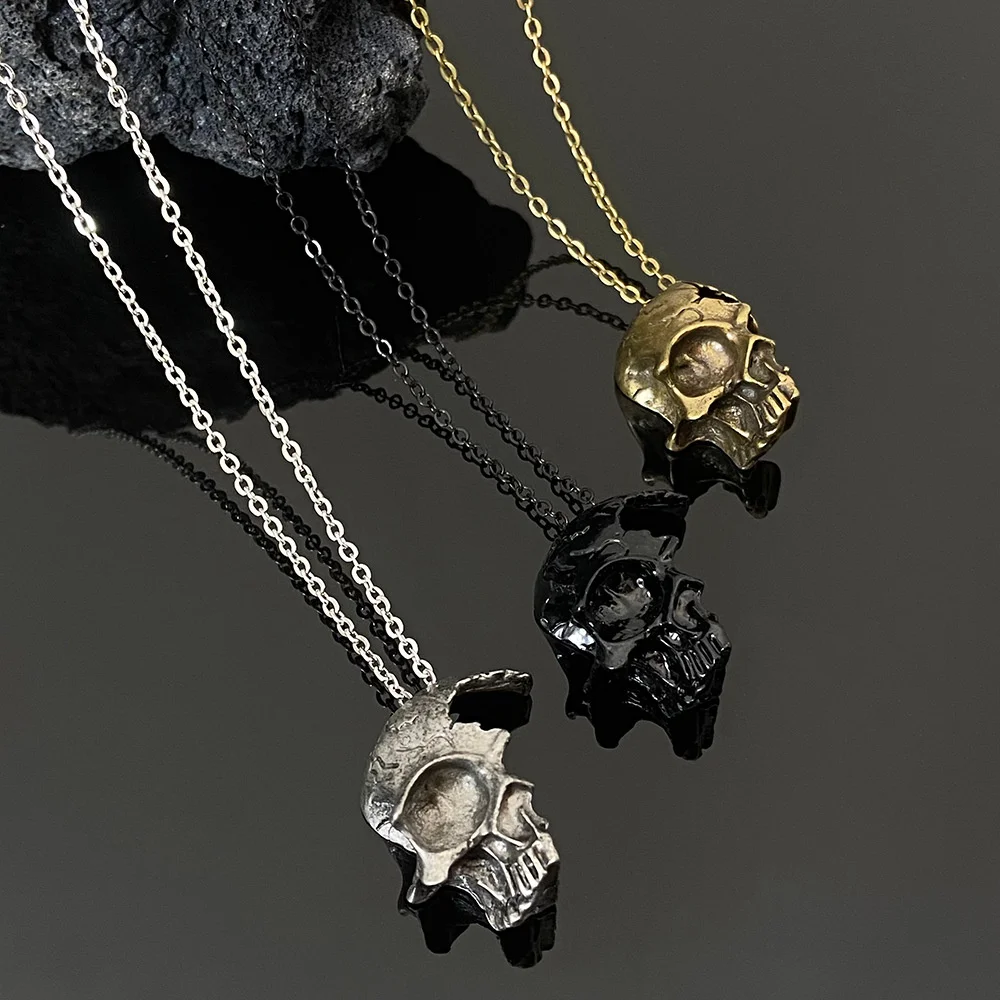The image showcases three intricately designed skull necklaces, each distinguished by its unique metallic finish and paired chain. Positioned against a solid black background, they collectively lean on a black, crystal-like lava rock located at the top left of the photo. The necklaces include a gold skull with a matching gold chain, a black skull with a corresponding black chain, and a silver skull with a silver chain. Each skull is artistically cracked and split in half, displaying only the left side with a singular eye socket, half of the nose cavity, and partial teeth. Notably, the top left section of each skull reveals a hole through the crack. The reflective dark gray surface beneath the necklaces accentuates the scene by mirroring their shadows, adding depth and contrast to the composition. The high-quality photograph meticulously captures these details, emphasizing the rugged elegance of the split skull design.